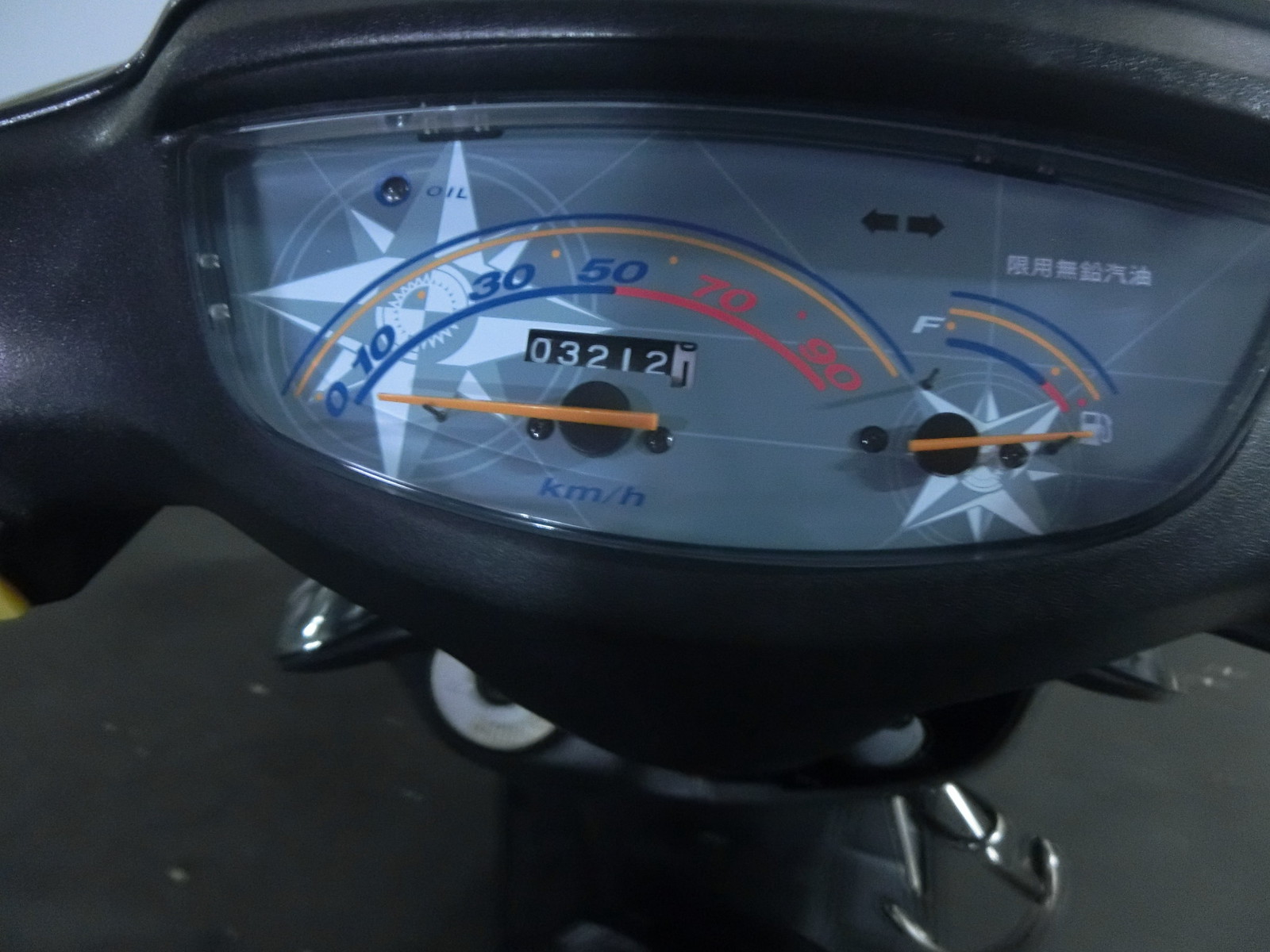This image portrays a dimly lit, close-up view of a motorcycle's speedometer and fuel gauge. The speedometer has a somewhat rounded, plasticky casing with gently curved edges, resembling the shape of a human eye. A clear plastic cover protects the front, through which several intricate details are visible. 

At the center of the speedometer, a yellow dial and a pointer stand out. The indicator sweeps across a light blue background marked with numerical values from 0 to 90, with increments of 10. The numbers 70 and 90 are displayed in red. The circular design is accentuated by curved yellow and blue lines that trace the arc of the dial. Below the dial, the text "KM/H" appears in blue.

Prominently featured in the background is an emblematic star with a gear in its center, reminiscent of a compass rose, adding a distinctive flair to the design. In the top left, a small indicator marked "oil" can be seen, while on the right side, a pair of arrows indicates the directions for the turn signals.

Adjacent to the speedometer, a similarly styled fuel gauge is visible. It shares the same blue, yellow, and blue color scheme. The gauge has a yellow pointer and features a gas tank symbol. The fuel levels are marked with "F" (Full) in blue on the left and a red section indicating lower fuel levels to the left of the gas pump symbol.